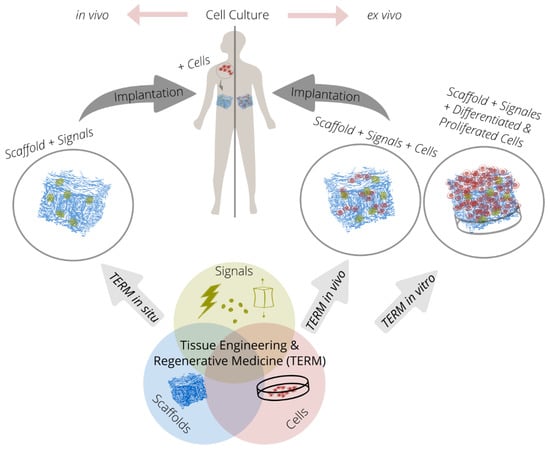This detailed scientific diagram illustrates the process of cell culture and its implications for tissue engineering and regenerative medicine (TERM). At the top, the diagram is labeled "cell culture," with arrows branching left and right, indicating "in vivo" on the left and "ex vivo" on the right. Below this label, an outline of a human body is depicted, with various images and arrows pointing towards the body to indicate the process of implantation.

In the central portion of the diagram, there are three distinct circles labeled "scaffold and signals" on the left, "scaffold, signals, and cells" on the right, and "scaffold, signals, and differentiated and proliferated cells" in the middle. These circles each contain diagrams showing what the cultured cells look like at different stages.

At the bottom, three interconnected circles represent the field of "tissue engineering and regenerative medicine," abbreviated as TERM. Arrows from these circles point upwards, suggesting a flow or progression towards the cell culture techniques described above.

The illustrations are drawn in a mix of styles, with some parts appearing computer-generated and others hand-drawn, utilizing colors such as blue, red, and yellow to differentiate between various components and stages of the process. This comprehensive diagram effectively conveys the flow from TERM to in vivo and ex vivo cell implantation, emphasizing the role of scaffold, signals, and cellular differentiation in creating viable tissue for medical purposes.